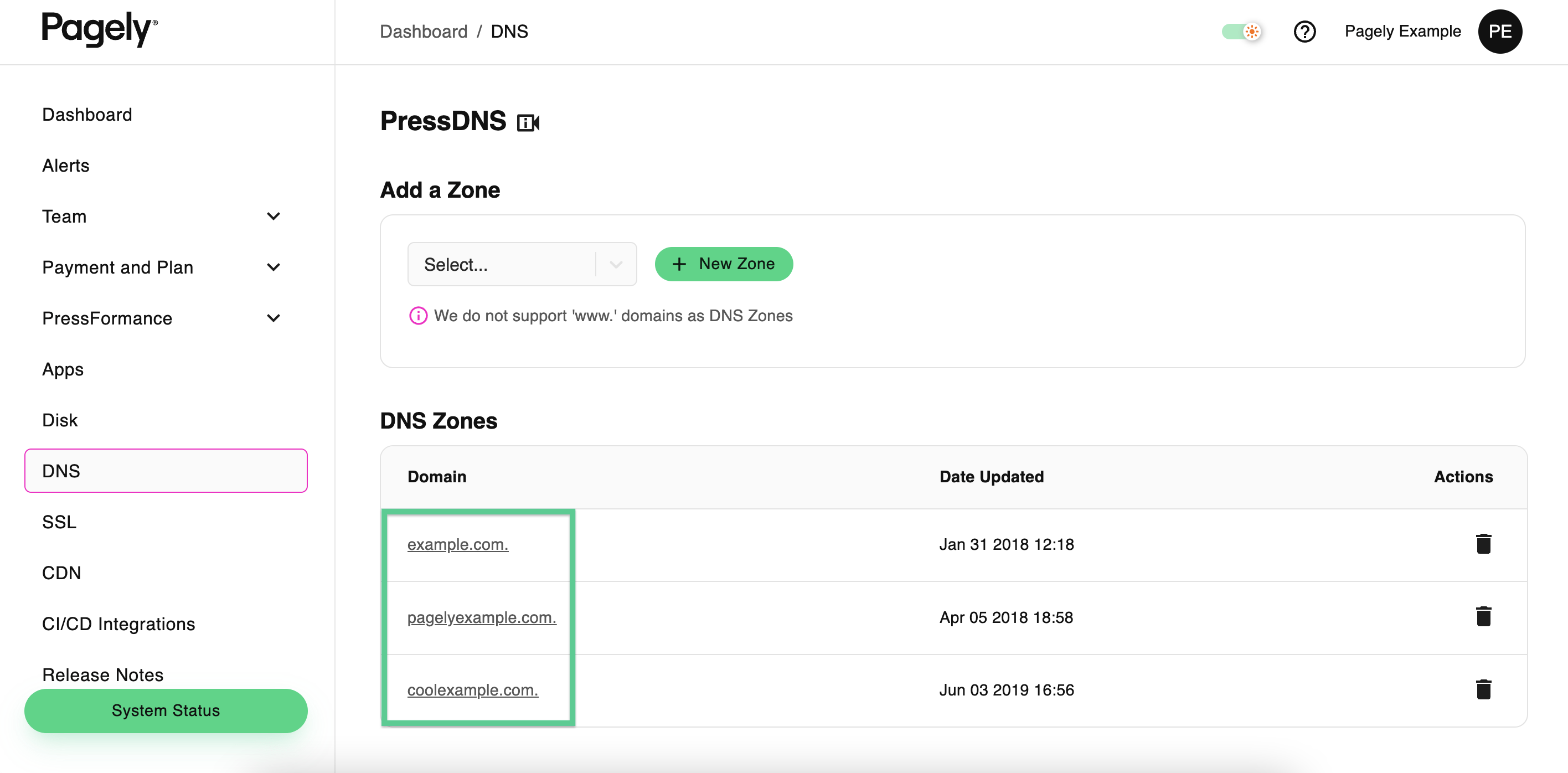In the top left corner of the image, the word "Pagely" is displayed in black text. To its right, "dashboard-DNS" is written. In the very top right corner, there is a circled question mark next to the text "Pagely example." Adjacent to this, there is a black circle containing the letters "PE." 

Beneath the "Pagely" logo on the far left, a navigational menu lists several items in descending order: "dashboard," "alerts," "team," "payment plan," "press formants," "apps," "disk," "DNS," "SSL," "CDN," "CI/CD integrations," "release notes," and "system status."

At the center of the image, under the "dashboard-DNS" heading, the words "press DNS" and "add a zone" are written. A dropdown box, labeled "select...," is visible, and to its right is a green button with a plus sign and the text "new zone."

Just below, there is a statement in small text indicating, "We do not support www.domains as DNS zones." 

Further down, there is a section titled "DNS zones" that includes headings for "domain" and a list of domain names: "example.com," "pagelyexample.com," and "poolexample.com." Each of these domains is marked with a green circle beside them. To the right of each domain, the date of upload is noted.